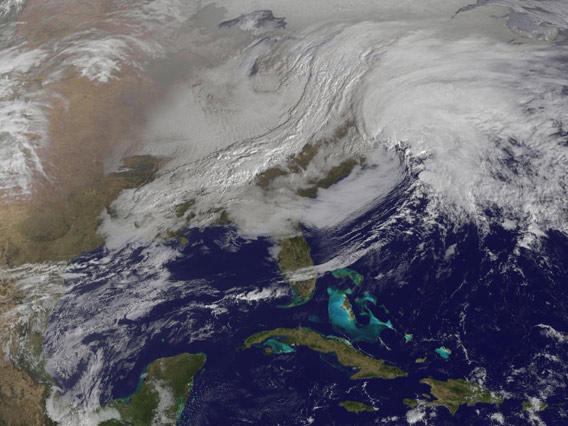A vibrant satellite photograph showcases a bird's-eye view of the southeastern United States, prominently featuring Florida and extending to the eastern seaboard. The deep blue waters of the Gulf of Mexico and the Atlantic Ocean frame the land, while various shades of green and brown depict the landscape. The image also highlights Cuba at the bottom and shows multiple islands with a mix of brown and green hues. The photograph is dominated by a large storm system, with wispy and fluffy white clouds blanketing much of the eastern U.S., stretching up to Michigan and the Great Lakes. There is a noticeable swirl pattern in the cloud cover, hinting at a significant weather event, possibly a hurricane, although it doesn't have the classical hurricane appearance. Snowy areas and wavy cloud formations add texture and depth to the scene, captured vividly from orbit.